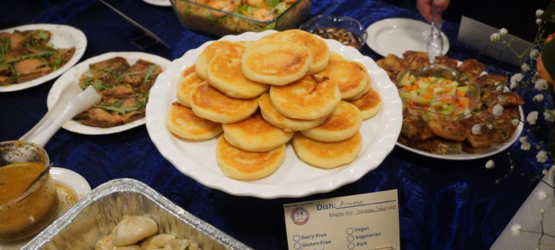In the center of the image, there is a white scallop-edged plate displaying a neatly stacked arrangement of small, thick pancakes that are golden brown, resembling round beige and cream-colored discs. In front of this central plate, at the bottom middle part of the picture, there is a white card with partially legible writing that reads "dish" and "made by" followed by an unreadable name. 

The scene is set on a blue velvet tablecloth, creating an elegant tablescape. Surrounding the central plate, various smaller plates and containers are arranged. To the bottom left, there is an aluminum pan containing white dumplings. To both the left and the right of the pancake plate, there are dishes featuring browned meats. Additionally, at the top right of the image, part of a person's hand is visible, holding a utensil and poised to dig into the food on the right.